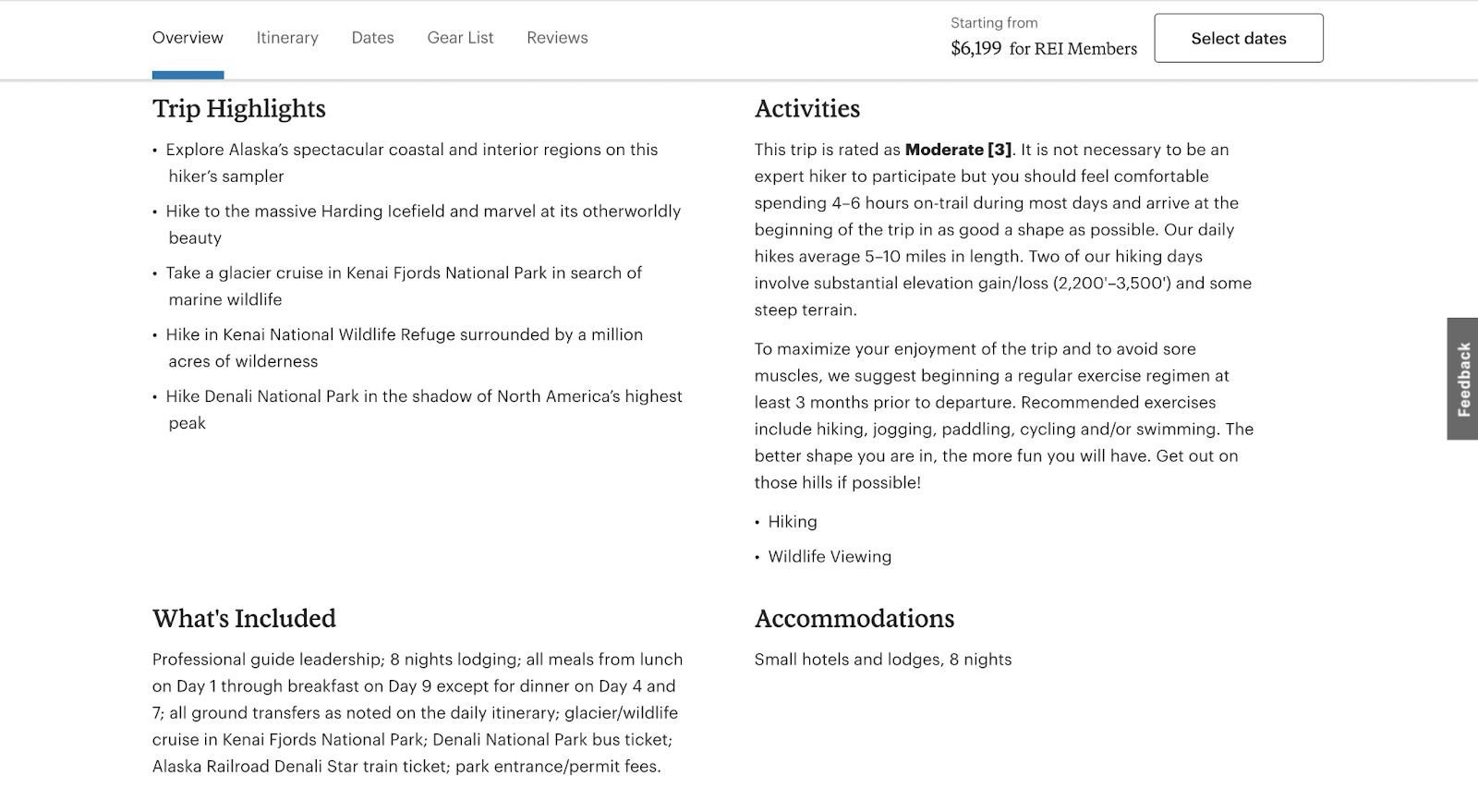**Image Description: Overview of an Alaska Hiking Adventure**

The image is a horizontal rectangle set against a white background, featuring a detailed layout of an Alaska hiking trip. At the top of the image, framed between two light gray lines, is the section labeled "Overview," highlighted with a turquoise underline and displayed in bold black font. Adjacent to this are additional categories written in unbolded black font: Itinerary, Dates, Gear List, and Reviews.

On the right side of the image, the text reads "Starting from," followed by a price, "$6,199," specifically for REI members. Beneath this is a box with the prompt "Select Dates."

To the left, a bold black headline reads "Trip Highlights," followed by descriptive bullet points in unbolded black text detailing the trip's features:
- Explore Alaska's spectacular coastal and interior regions on this hiker sampler.
- Hike to the massive Harding Ice Field and marvel at its otherworldly beauty.
- Take a glacier cruise in Kenai Fjords National Park in search of marine wildlife.
- Hike in Kenai National Wildlife Refuge, surrounded by a million acres of wilderness.
- Hike Denali National Park in the shadow of North America's highest peak.

In a second column on the right, a bold black heading "Activities" is followed by regular black text stating that the trip is rated as "Moderate" (indicated by a number 3 in brackets). It clarifies that while expertise in hiking is not required, participants should be comfortable with spending 4 to 6 hours on the trail and be in good physical condition at the trip's start. The daily hikes average 5 to 10 miles, with some days involving significant elevation changes (2,200 to 3,500 feet) and steep terrain.

An additional paragraph suggests starting a regular exercise regimen at least three months before the departure date, recommending activities such as hiking, jogging, paddling, cycling, and swimming to enhance enjoyment of the trip.

Further, there are bullet points highlighting activities:
- Hiking
- Wildlife Viewing

To the right of these sections is a vertical gray box containing the word "Feedback" in white.

Under "Activities," the bold black heading "Accommodations" reveals that the trip includes stays in small hotels and lodges for eight nights.

Back on the left side of the page, the bold black heading "What's Included" lists the following items in regular black font:
- Professional guide leadership
- Eight nights lodging
- All meals from lunch on day one through breakfast on day nine, except for dinner on day four and seven
- All ground transfers as noted on the daily itinerary
- Glacier/Wildlife cruise in Kenai Fjords National Park
- Denali National Park bus ticket
- Alaska Railroad Denali Star train ticket
- Park entrance/permit fees